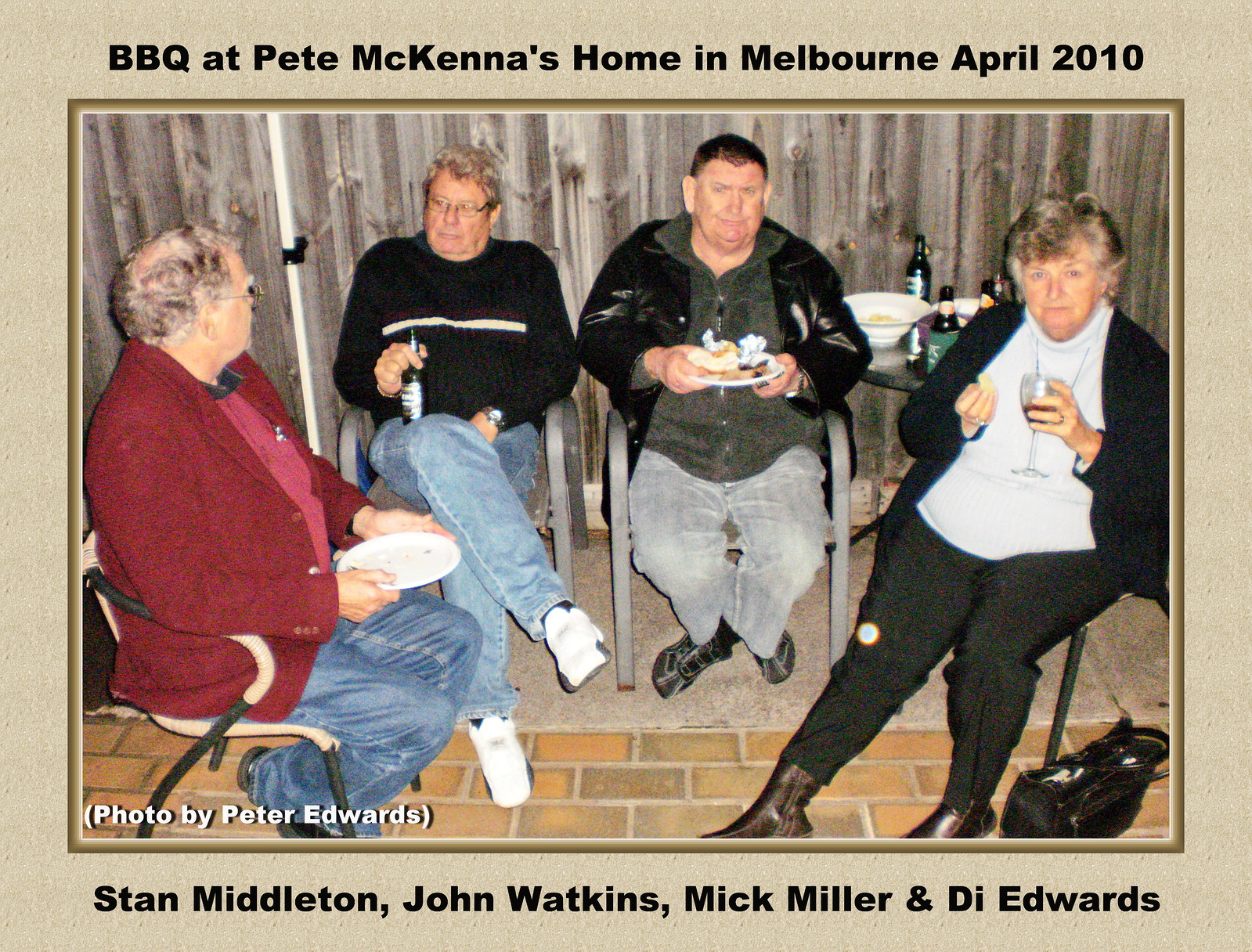The photograph features a beige or tannish-colored border around it, set within a framed, possibly gold-matted setting. At the top, the caption in black letters reads, "Barbecue at Pete McKenna's home in Melbourne, April 2010." The image showcases four individuals on a brick patio in outdoor chairs, positioned against a wooden fence. From left to right, the names at the bottom of the photo indicate, "Stan Middleton, John Watkins, Mick Miller, and Di Edwards." 

Stan Middleton, on the far left, is an older man with balding gray hair, wearing a red jacket and jeans; he appears to be looking towards John Watkins. John, the second person, is middle-aged, dressed in a black sweater, and holds a beer on his lap while looking off to the side. Centrally seated is Mick Miller, sporting a black jacket over a gray sweater, short hair, and a grumpy expression while holding a plate of food. Di Edwards, on the far right, wears a dark cardigan over a white shirt with black pants and has short gray hair; she looks directly at the camera while holding a drink. A side table in the corner with drinks and bowls supports the social ambiance. Additionally, a white watermark on the bottom left identifies the photo credit: "Photo by Peter Edwards."